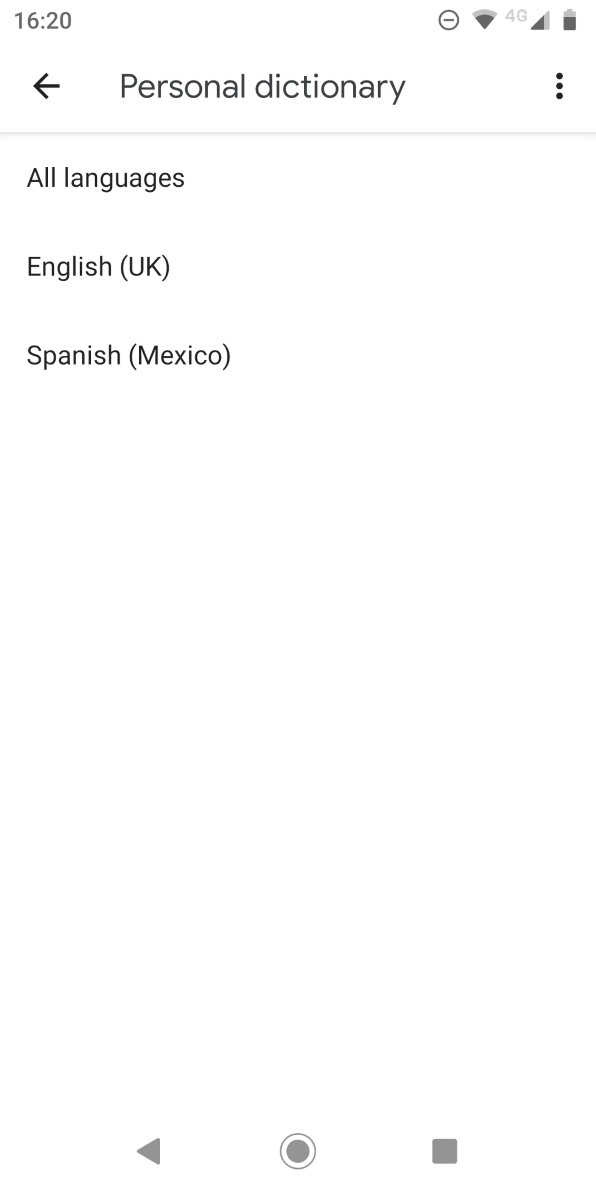The screenshot depicts a phone's settings menu. At the top-left corner, the time is displayed as 16:20. In the top-right corner, a series of icons appear: a circular icon with a line through it, a Wi-Fi icon, a cell phone signal indicator showing a nearly full 4G signal (grayed out), and a battery icon indicating approximately 60% charge.

The main heading, "Personal dictionary," is prominently displayed, with "Personal" capitalized and "dictionary" in lowercase. To the left of the heading is a left-facing arrow, and to the right are three vertical dots indicating a menu.

Below the heading is a light gray line break. Underneath this line, the text "All languages" appears in black. Subsequent lines list individual languages: "English (UK)" followed by "Spanish (Mexico)."

The background of the screenshot is entirely white. At the bottom of the screenshot, there are three gray icons. On the left is a triangle pointing left, resembling a reverse play button. In the center is a filled gray circle with a white border, possibly indicating a record function. To the right is a gray square, similar to a stop button. The purpose of these icons in relation to the "Personal dictionary" setting is unclear.